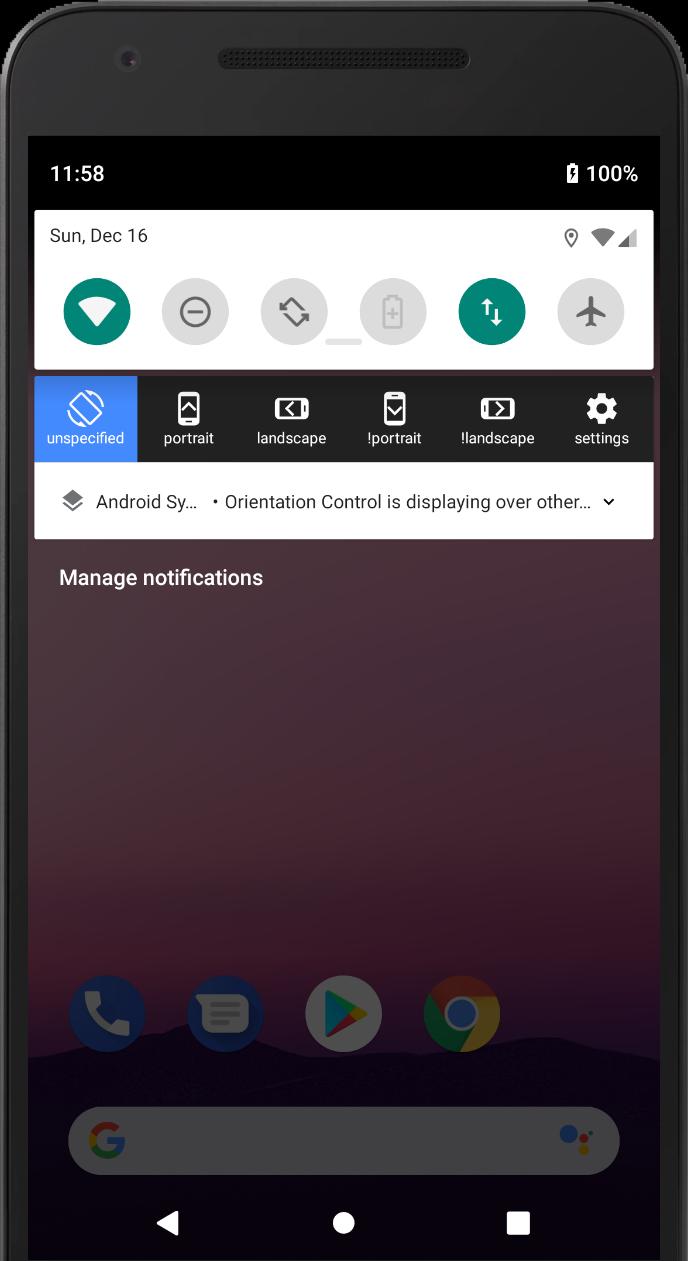The screenshot displays a smartphone interface with intricate details. In the top-left corner, the current time is 11:58 AM. Moving to the top-right corner, the battery level is fully charged at 100%. Just beneath, the date is specified as Sunday, December 16th. Adjacent to the date, the Wi-Fi signal is strong and the location services are enabled.

Below this information, a row of six circular icons is visible. The first icon, representing Wi-Fi, is activated and highlighted in green. The subsequent three icons include an unspecified battery-related symbol, another icon with arrows pointing up and down (potentially indicating data transfer), and an airplane mode icon, which is currently inactive. Among these, only the Wi-Fi and the up-and-down arrows are activated.

Further down, there are additional controls for screen orientation. The labels are: "portrait," "landscape," "portrait" again, and "landscape" once more. An unspecified option is also highlighted, likely indicating the current setting. Below these controls, the text "Android SY" appears, followed by the phrase "orientation controls displayed over other," accompanied by a downward-facing caret symbol suggesting more information is available. Finally, at the bottom, there's an option labeled "Manage notifications," hinting at further customization settings.